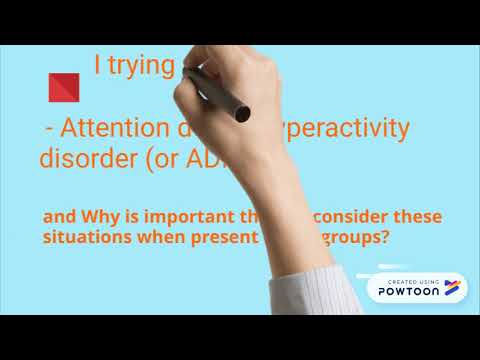In the image, we see a graphical design featuring a Caucasian woman's extended forearm and hand, holding a thick pen positioned as though she is actively writing on a light blue background. The hand starts from the bottom right edge and reaches towards the top center of the image. At the top center, in orange text, there are the words "I trying," which align with the pen's tip. Below this, some of the text is obscured by the hand, making parts of the sentence incomplete. The visible text reads: "attention," followed by "per activity disorder, or AD," and continues with "and why it is important to consider these situations when present, groups?" The image is framed by black header and footer bars, adding a structured look to the otherwise minimalist design. Additionally, a red square is positioned in the upper left corner, contrasting with the light blue background. In the lower right corner, within a white oval speech bubble, it states, "created using Powtoon" in blue writing. This detailed composition suggests an intentional design element, possibly for a presentation or educational content.